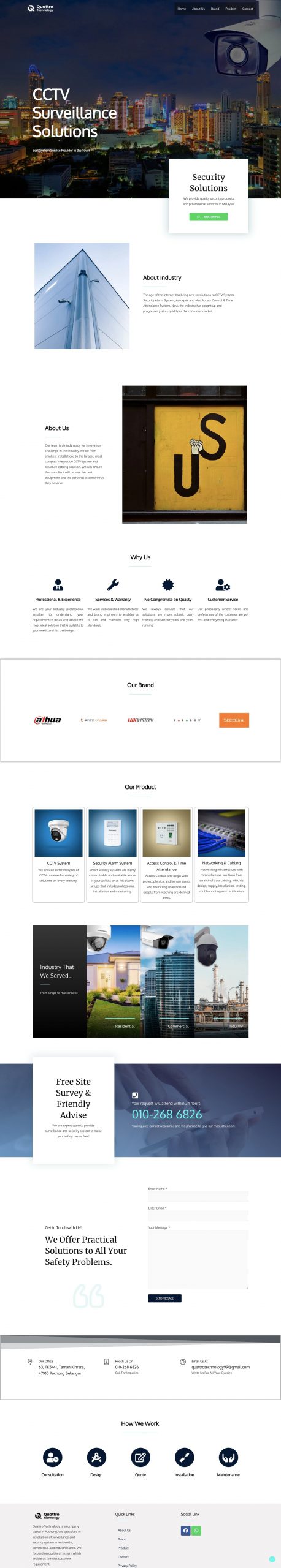This is a detailed caption for an intricate screenshot of a smartphone interface. The image showcases various sections, colors, and textual elements, enhancing the complexity and emphasizing the wide array of features displayed. Here's the refined and highly detailed caption:

---

The screenshot displays a smartphone interface characterized by its multifaceted and vibrant layout. At the top of the screen, a dark section features a city skyline rendered in silhouette, suggesting an urban environment. On the left side of this section, "CCTV Surveillance Substations" is written in bold white text. Opposite this, on the right, is a white box containing some black text that is too small to discern clearly. Beneath this box runs a green bar, followed by another white box below.

This second white box is notable for containing a blue triangle pointing upwards, bordered by several blue lines. These lines curve dynamically—some bending to the left, others to the right, and some extending straight upwards. Adjacent to these blue lines is more black text, again too minute to read clearly.

Further down, the interface transitions to a black box. Within the bottom right corner of this section, there is a brown box emblazoned with the letters "U" and "S," where the "U" is positioned lower than the "S." Positioned to the left of this brown box is additional small black text, which remains illegible.

Below this, there are three sets of black text, each too small to read, each preceded by a tiny black icon that is indistinguishable. Directly beneath these elements is another white box featuring five distinct links. These links exhibit varying colors: the leftmost is black, the second is gray, the third (in the middle) is a blend of black, and the fourth has a gray and orange-colored shadow.

Progressing downward, four boxed icons are visible. The first, on the left, is a blue box with a white printer icon. Next to it is another blue box containing a white page icon. Adjacent is a gold-colored box with a white phone icon. The final box is a dark blue, and each of these boxes has supplementary small black text underneath them, which is too small to decipher.

Continuing down, a long rectangle is present, transitioning from black on the left to a depiction of city skylines towards the right. Below this is another lengthy black rectangle, this time fading from blue at the top to a lighter blue at the bottom. Towards the right of this section exists a white square with minuscule black text. Following this, another white section appears, containing a long black line underneath.

The interface rounds off with several additional elements: a gray section with a long gray line extends below some text, along with a series of five small oval-shaped buttons with text too small to make out. Further below, the bottommost part of the screen appears as a long gray section with multiple lines of black text on the left. The center features another set of lines, while towards the right, black text rests above a pair of buttons — one blue and the other light green — both of which bear inscriptions too small to read.

---

This caption meticulously details each element within the screenshot, providing a comprehensive and vivid description of the smartphone interface.